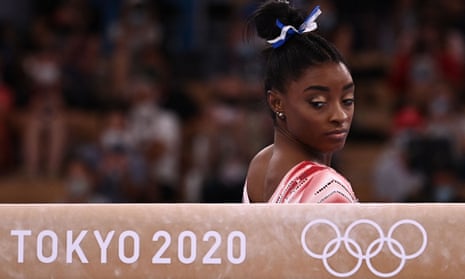This landscape-oriented color photograph captures a significant moment at the Tokyo 2020 Olympics, featuring the renowned gymnast Simone Biles. Positioned slightly to the right of center, Simone stands with her body facing right, her head turned back over her right shoulder, providing a three-quarter view of her face. She wears a red, pink, white, and black leotard with a scoop neckline in the back, and her hair is neatly pulled up into a bun adorned with a white ribbon. Small gold stud earrings add a subtle touch of elegance.

Simone's expression is serious as she looks slightly downward, seemingly focused and possibly about to commence her routine. Despite the blurred backdrop of spectators in the bleachers, she remains the unmistakable focal point of the image. The photograph is framed by a wide horizontal beige banner at the bottom. In white text, the banner reads "Tokyo 2020" on the left, and to the right, it features the iconic five interlocking Olympic rings. The image is a vivid representation of the moment, blending photographic realism with representational art to highlight the athlete's poised readiness amidst the grandeur of the Olympic Games.